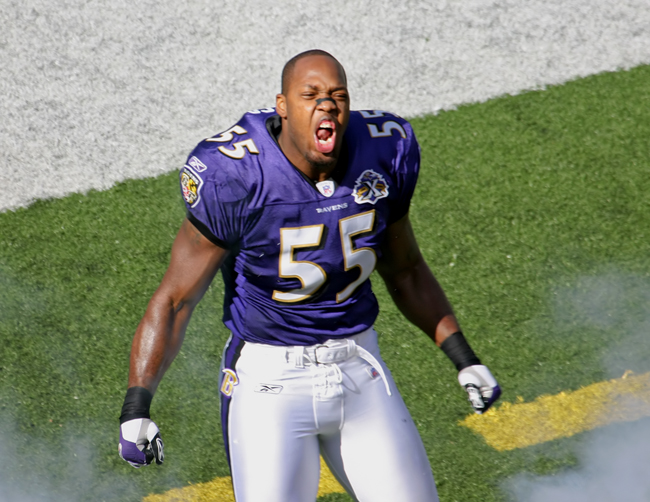The photograph captures an intense moment as a football player, predominantly clad in a purple jersey and white pants, celebrates or shouts energetically. His uniform features distinctive details: the purple jersey emblazoned with the number 55, highlighted by a yellow border on both the front and the shoulders, and "Ravens" inscribed in white close to the neckline. The player's white pants, adorned with purple stripes and a gold 'B' near the waistline, are secured by a white belt with a silver buckle. His fists, clenched tightly in white and purple gloves, underscore his fervor. The image, framed from above his knees to the top of his head, reveals his expressive face with a wide-open mouth and squinted eyes. Standing directly in the center of a grassy, painted football field under the bright daylight, the player's short black hair and muscular build are also noticeable, making for a powerful and dynamic portrayal.